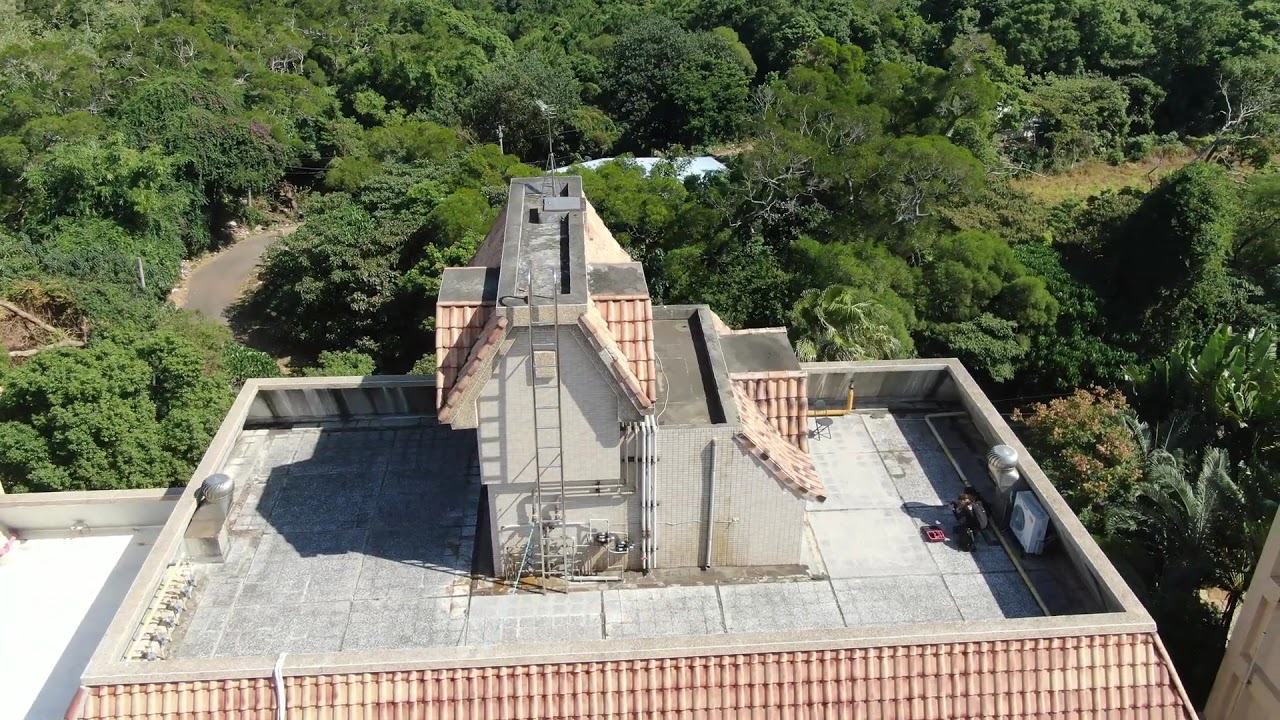The image shows an aerial view of the rooftop of a tall building, possibly a castle or a large house. The roof is primarily covered in pink terracotta tiles with a flat section made of gray concrete slabs. In the center of the roof stands a small turret or structure, potentially an elevator shaft or stairway access. The rooftop features several ladders, air conditioning units, fans, and an antenna, indicating it's a functional space. On the right side of the roof, a man in dark clothing, possibly with a black backpack, is squatting and either working or taking pictures. His shadow is clearly visible on the sunny rooftop. Below the rooftop, there is a dense expanse of trees, including a tropical one, extending out of the frame. The trees crowd the area so densely that the ground is barely visible, contributing to the secluded and natural setting of the building. In the background, another building's rooftop with white elements and radio towers is faintly visible amidst the foliage.